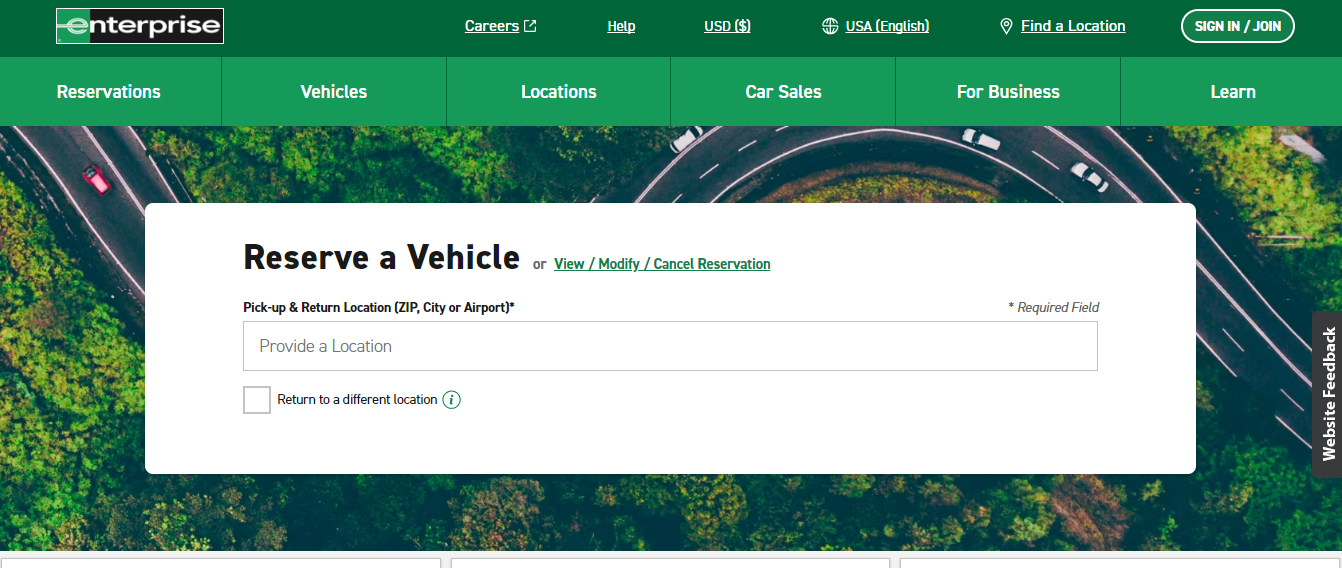The image depicts the homepage of the popular car rental website, Enterprise. The background features two shades of green, creating a distinct and recognizable brand theme. At the top, there's a rectangular bar with the Enterprise logo. Along this bar, several navigation buttons are clearly labeled: "Careers," "Help," "USD Money," "USA English," and "Find a Location," with an oval button on the right labeled "Sign In/Join."

Below this navigation bar, a series of options are presented for users to navigate different sections of the website: "Reservations," "Vehicles," "Locations," "Car Sales," "For Business," and "Learn."

Centrally placed over a captivating aerial image, there's a functional banner where users can reserve a vehicle. In bold, prominent text, it reads: "Reserve a Vehicle or View, Modify, Cancel Reservation." Beneath this, there are fields for "Pick-up and Return Location," with instruction to enter a zip code, city, or airport. Additionally, a checkbox option labeled "Return to a Different Location" is available, accompanied by a small, green circle with an "i" for information.

The background image behind the reservation banner is a scenic photograph captured from a drone or an airplane, showing a winding black asphalt road with white lane markings. A couple of white cars and a solitary red car are visible on the road, all surrounded by lush green trees, creating a visually appealing and engaging interface.